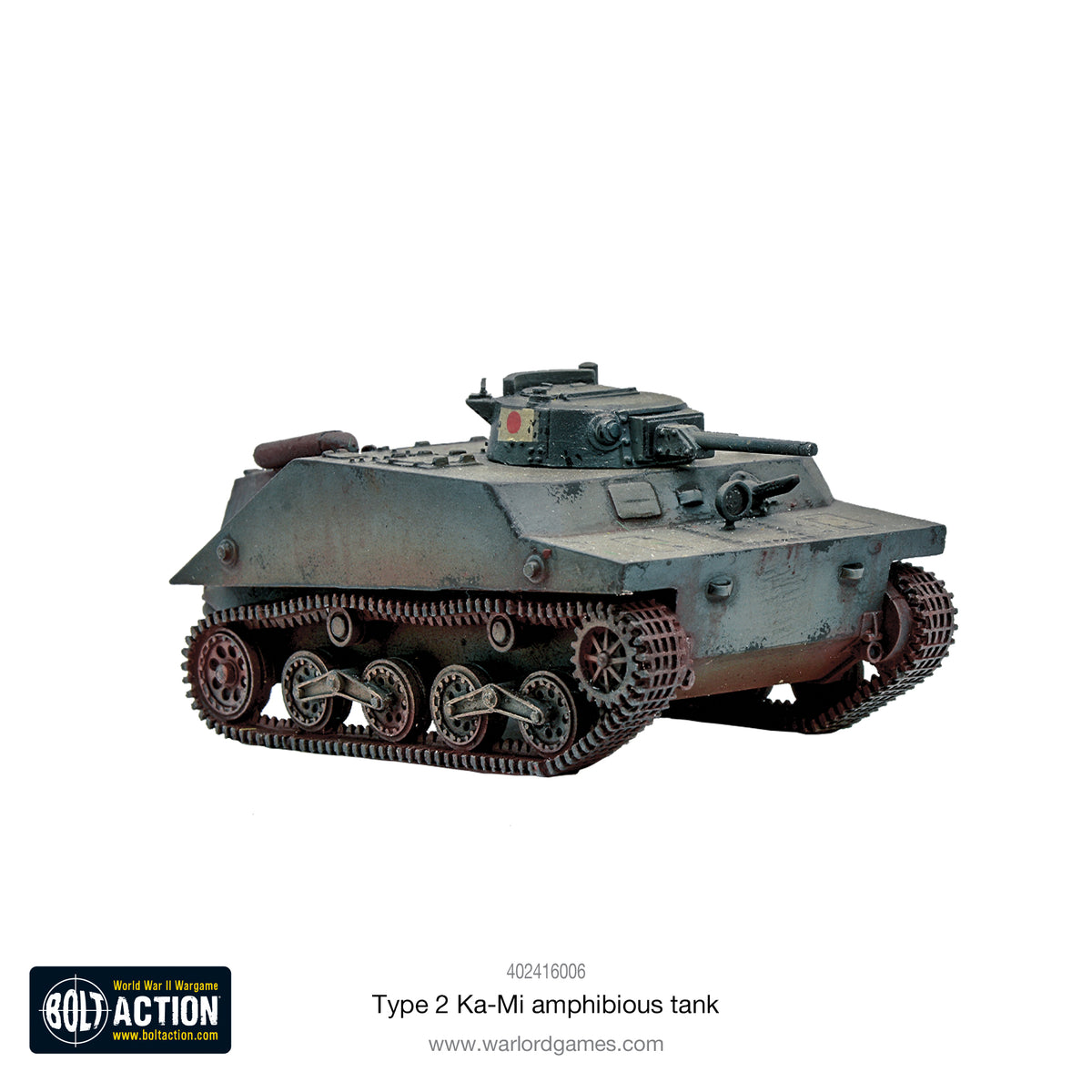This image depicts a detailed model of a Type 2 Ka-Mi Amphibious Tank from WWII, showcasing a greenish-gray color with patches of patina and rust on the treads and body. The tank is oriented to the right and features a short-barrel gun on top, along with a small Japanese flag consisting of a red circle on a white background near the opening on the top portion. The model includes six visible gear-like wheels on one side, a prominent chain for terrain navigation, and various signs of wear, giving it a realistic and battle-worn appearance. Text at the bottom center of the image reads "402416006 Type 2 Ka-Mi Amphibious Tank www.warlordgames.com," while the lower left corner displays "WWIIWARGAMEBOLTACTION.COM" and a logo with "Actable2Action.com."